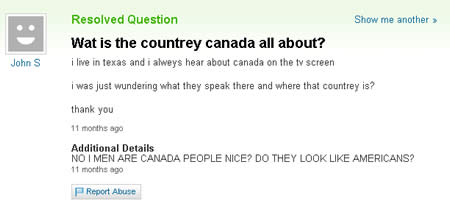This image is a screenshot from a web page, featuring a gradient background that transitions from light green at the top to white further down. 

In the top left corner, there is a light gray outlined square with a white interior. Within this white square is a smaller gray square showing a simple emoticon with two circles for eyes and a smiling mouth. Beneath this icon, the text "John S" is displayed in blue with a capital "J" and a capital "S".

To the right of this, in lime green text with capitalized initials, it reads, "Resolved Question." Positioned to the far right is the phrase "Show me another," with a right arrow next to it. The initial "S" is capitalized and the text is blue.

Further down, in bold black print, the text reads, "What is the country Canada all about?" The word "country" is misspelled as "countrey." Below this question, additional text states, "I live in Texas, and I always hear about Canada on the TV screen. I was just wondering what they speak there, and where that country is." Here, "country" is misspelled again, and "wondering" is incorrectly spelled as "wundrang."

Continuing below, the post includes "Thank you," followed by a timestamp from "11 months ago." There’s a section labeled "Additional Details," presented in an older, more formal print with capitalized initials "A" and "D." This section says, "No, I meant, Are Canada people nice? Do they look like Americans?" in all capital letters. This addendum is also timestamped from "11 months ago."

Towards the bottom right, there is a small button with the text "Report abuse" accompanied by a blue flag icon. The text on this button is also blue.